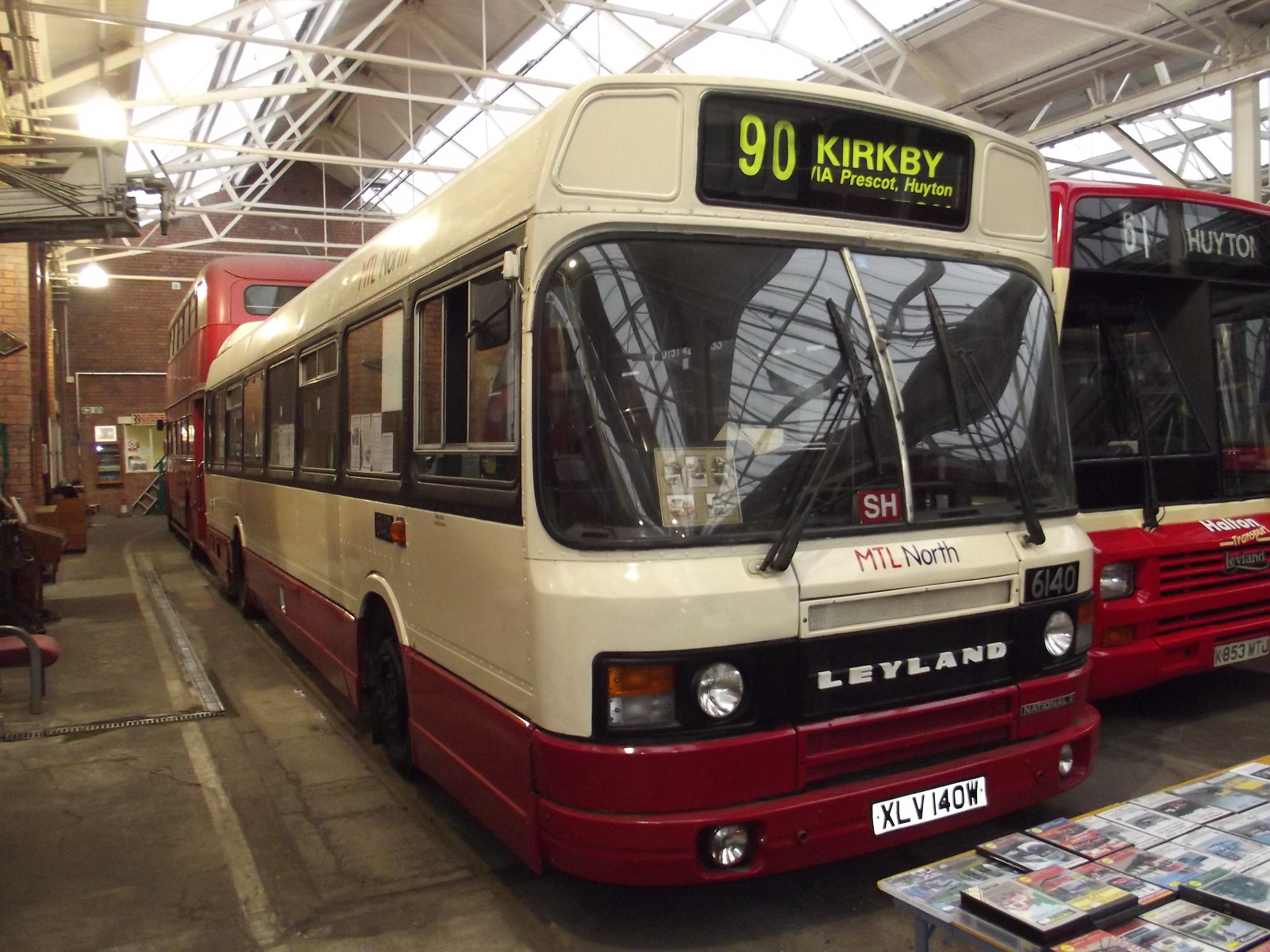The image showcases a garage with three city buses parked inside. The garage itself has a brick construction with a metal ceiling outfitted with skylights, and the buses are parked on a cement floor. In the foreground, there is an older Leyland bus, likely from the 1970s or early 1980s, marked as the number 90 bus with the route "Kirkby Prescott Whiten" displayed across the top sign. This bus is predominantly white with dark red trim along the bottom. The large windshield prominently features the letters "SH" in white on a red background, and below it, between the headlights, the name "Leyland" is inscribed on a black background. Its license plate reads "XLV40W". Directly to the right of this bus is another red bus with beige trim, marked "Whiten" at the top. In the far rear, a double-decker red bus can be seen. The ceiling structure of the garage includes metal scaffolding, reinforcing the industrial look of the space.